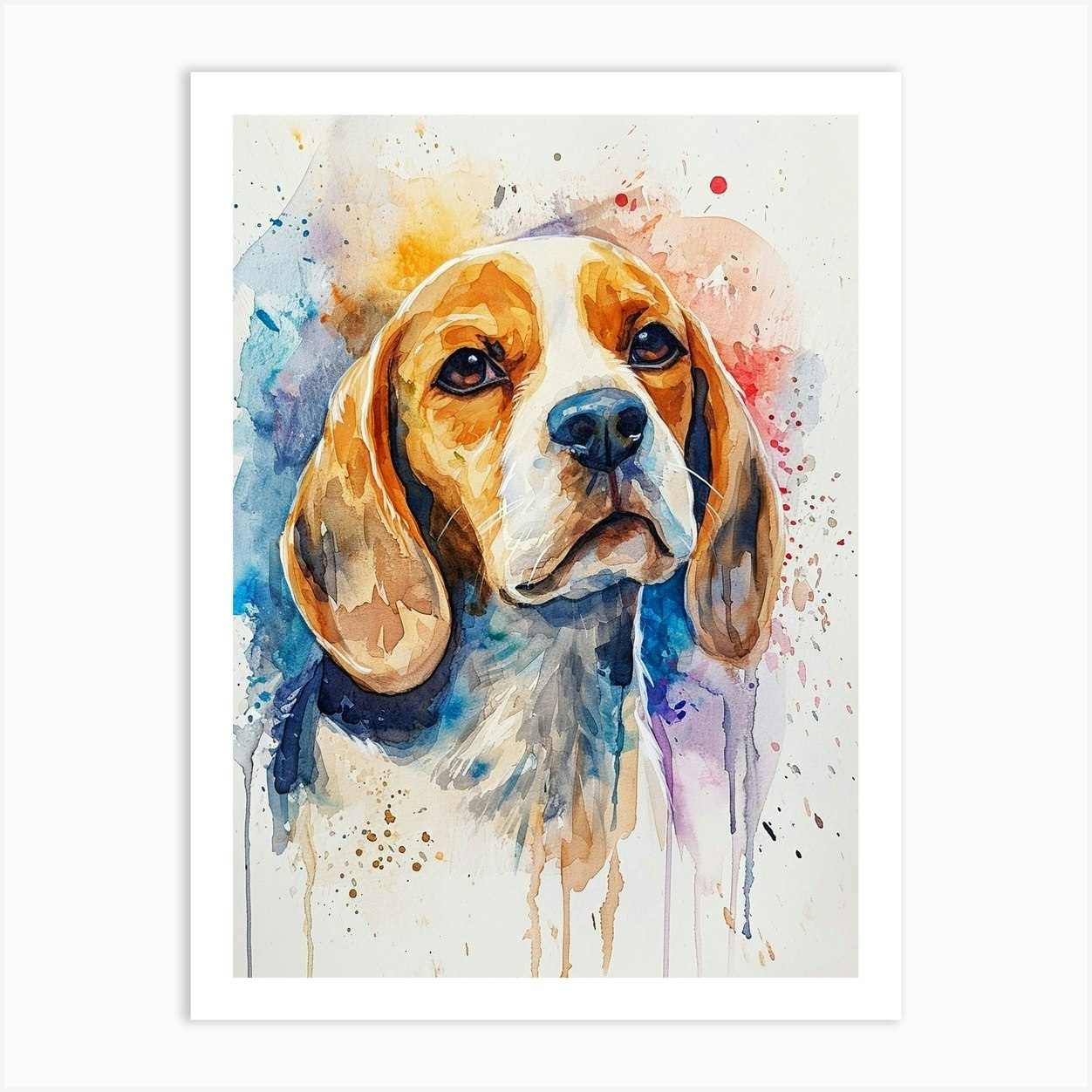The image depicts a detailed watercolor painting of a beagle, centrally placed on a vertically oriented rectangular canvas with a white border and a subtle drop shadow, suggesting it's positioned on a light gray surface. The beagle's face is well-defined, featuring big, deep brown eyes, a black nose, and a white snout extending up between the eyes to the top of the head. The fur around the eyes and the droopy ears is a blend of golden brown, orange, and yellow hues, with hints of gray shading for depth. Only a bit of the dog's body is visible, mostly fading into abstract art. Surrounding the beagle's head is a vibrant array of watercolor splashes that drip downwards, punctuated with blobs and speckles of red, purple, blue, and yellow paint, adding a dynamic background to the serene canine portrait.